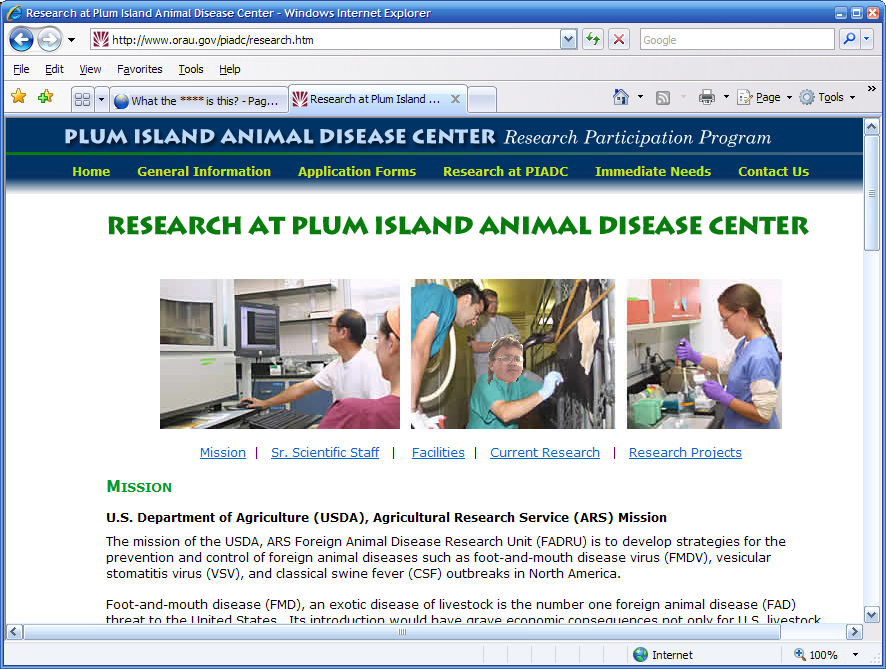In an Internet Explorer browser window, a user is currently viewing a website called urau.gov. The browser shows two open tabs; the first tab intriguingly titled "What the blank is this?" with the content of that page unknown. The primary focus is on the second tab displaying a page about the Research at Plum Island Animal Disease Center. The page is rich with information and features images of people working in a laboratory setting. The highlighted section states the mission of the U.S. Department of Agriculture's Agricultural Research Service (USDA ARS) Foreign Animal Disease Research Unit. The mission aims to develop strategies for the prevention and control of foreign animal diseases, including foot-and-mouth disease virus, vesicular stomatitis virus, and classical swine flu outbreaks in North America. The webpage includes several links for more detailed sections such as Senior Scientific Staff, Facilities, Current Research, and Research Projects. Additional navigation options near the top of the page offer links to General Information, Application Forms, Research, Immediate Needs, and Contact Us. The distinct Internet Explorer interface is visible at the top of the screen.